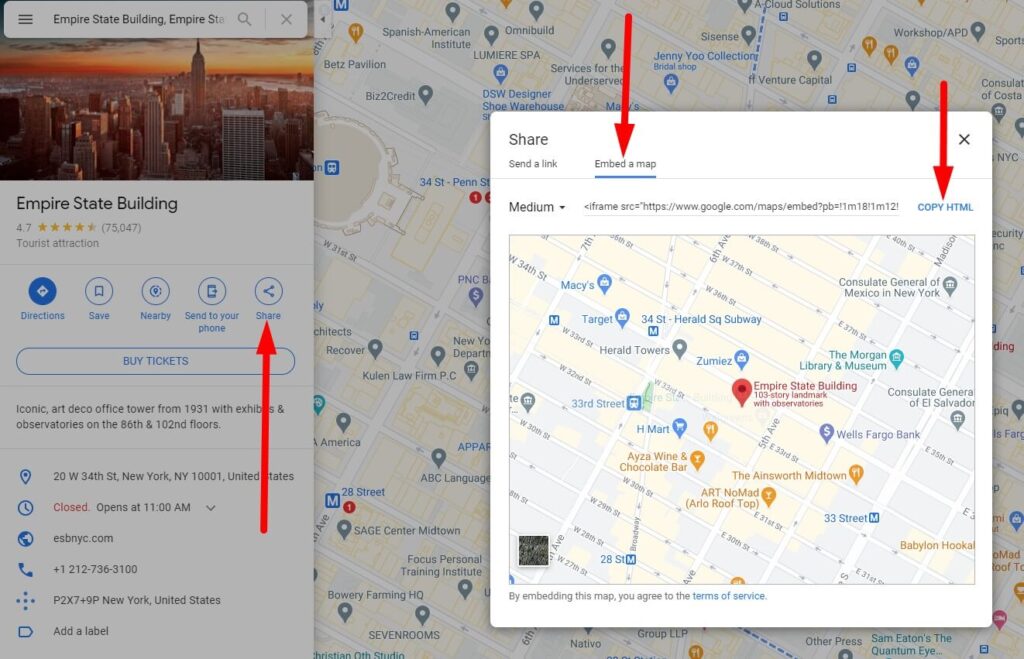This is a detailed screenshot of Google Maps showing the search results for the Empire State Building. The search bar located on the left-hand side displays "Empire State Building, Empire State," accompanied by an aerial image of the building during sunset or sunrise. Below this, the Empire State Building's profile indicates a rating of 4.7 stars from 75,047 reviews, categorizing it as a tourist attraction. Several options are listed: directions, save, nearby, send to your phone, and share.

Three distinct red arrows highlight different areas of this screenshot. The first arrow points to the 'Share' button, triggering a pop-up window on the right side of the screen. This window offers two options: 'Send a link' and 'Embed a map'. The second arrow directs attention to the dropdown menu in the 'Embed a map' section, which has 'Medium' selected. The final red arrow points towards the 'Copy HTML' button, which is adjacent to the selected size dropdown. Below the dropdown is a text box containing the HTML code, available for copying. The overall layout includes a pop-out map displaying the specific location of the Empire State Building.